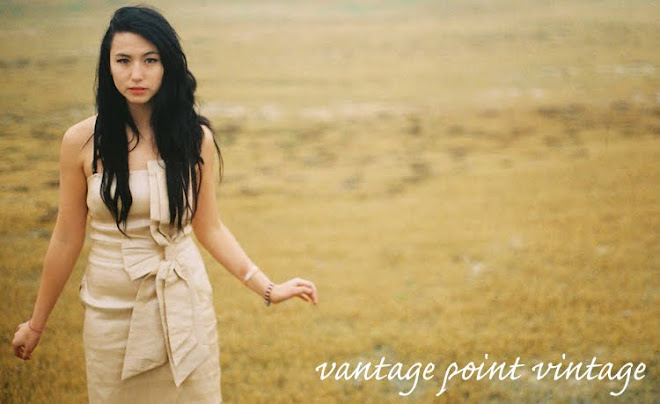In the foreground of the image, a woman is captured walking in a sprawling, tan and yellow grassy field that fades into the horizon. She has long black hair cascading down her shoulders and her lips are a noticeable red, adding contrast to her fair complexion. She is dressed in an off-white, strapless dress with a notable bow at the waist, reminiscent of elegant bridesmaid attire. Her arms, adorned with a bracelet on her left wrist, hang by her sides, slightly tilted outward. The background is a blur of tan and light brown, enhancing the model’s prominence in the image. In the bottom right corner of the photo, the cursive text "Vantage Point Vintage" is inscribed. The overall color palette includes shades of black, white, tan, brown, and red, amplifying the vintage aesthetic of the photograph.